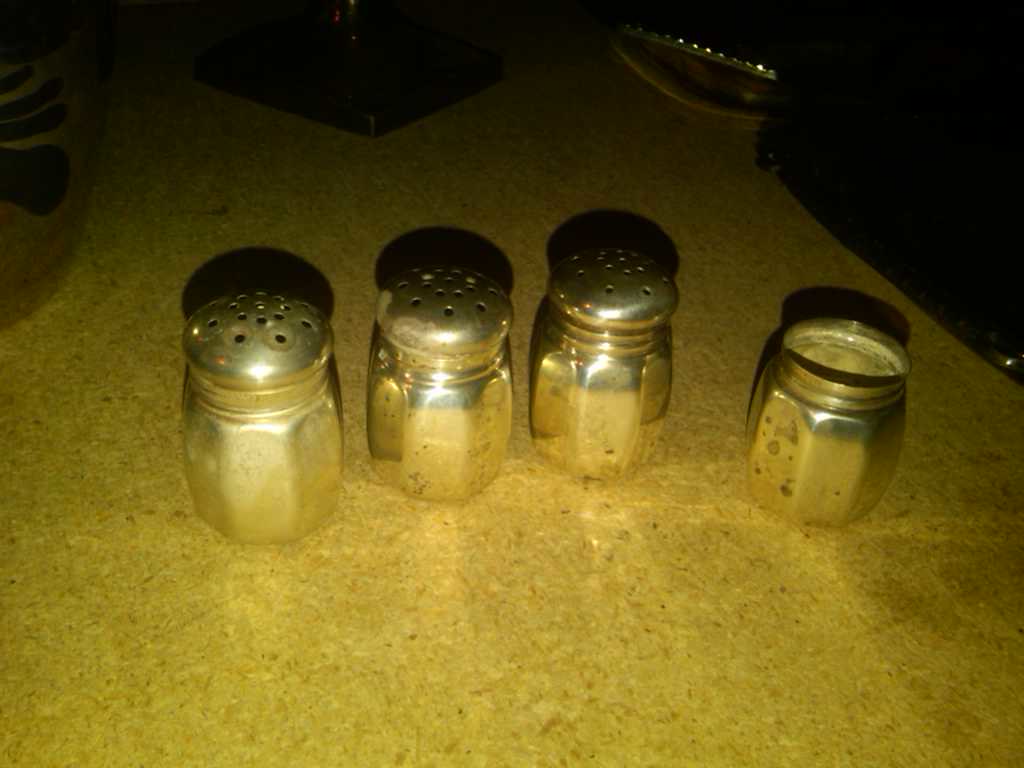The photograph captures a dimly lit kitchen scene, with the focus on an old Formica countertop in the center bottom of the image. On the countertop, there are four glass jars arranged in a slight line. These jars resemble classic diner salt and pepper shakers with metal tops. Three of the jars have perforated metal lids and are filled with a dark substance, likely pepper, while the fourth jar, on the far right, lacks a lid. This lidless jar exposes the contents inside. The poor lighting causes the jars to cast distinct shadows behind them. In the upper right-hand corner of the photo, a dark, nearly black area is visible, and a hint of a shoe appears. The background remains obscure due to the low light, adding an air of mystery to the setting.